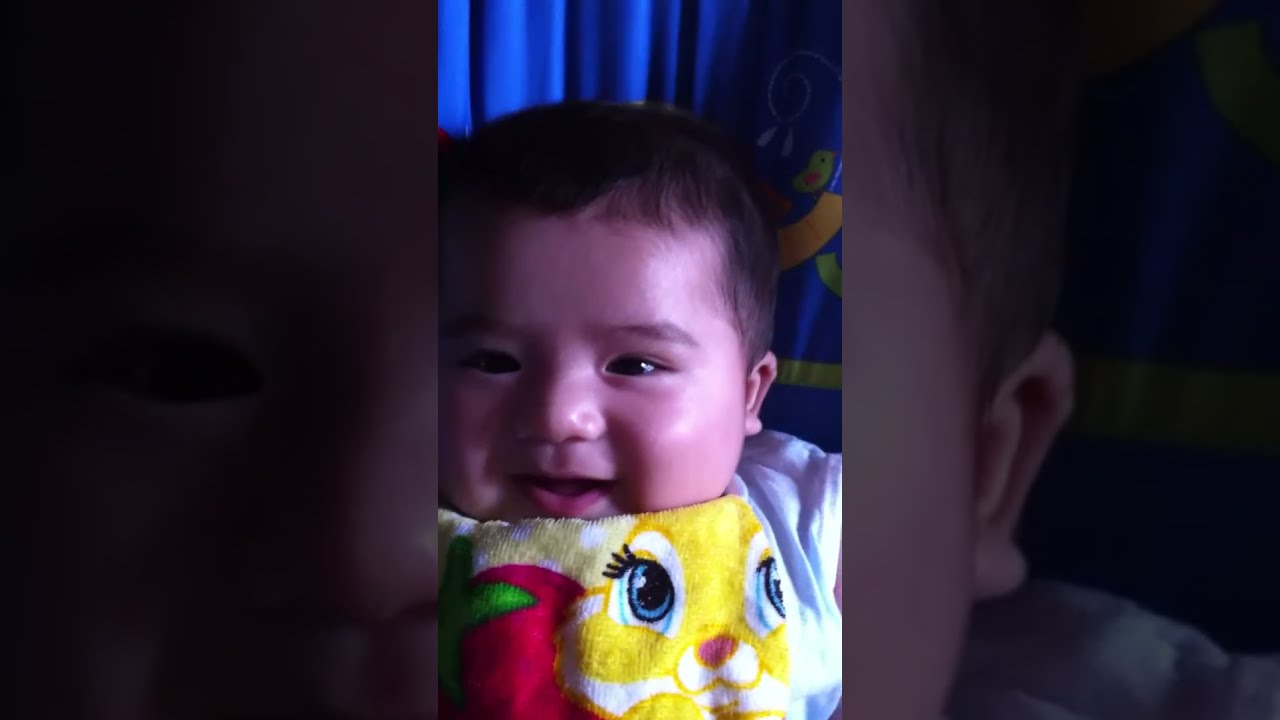This detailed image consists of three panels. The central panel, in portrait orientation, features a close-up, color photograph of a young infant boy, possibly around four or five months old. He has dark hair and skin, and he is beaming with a big smile. The infant is oriented slightly to the left of the center, dressed in a colorful bib adorned with a yellow bunny rabbit with large blue eyes and a red tomato or strawberry to the left. He seems to be either sitting up in a high chair or lying down with a piece of clothing—possibly fur or cloth—underneath his neck, obscuring his chin. In the background, there is a blue curtain, suggesting a studio setting, and additional blue and yellow elements are visible in the right corner.

The two outer panels, slightly larger and in landscape orientation, are underexposed, darkened blowups of the central photograph. These panels display the right and left halves of the central image, emphasizing the photo's realism and representationalism. The detailed background of blue drapes and the close-up perspective in the center photo create a striking, intimate portrait of the smiling infant.